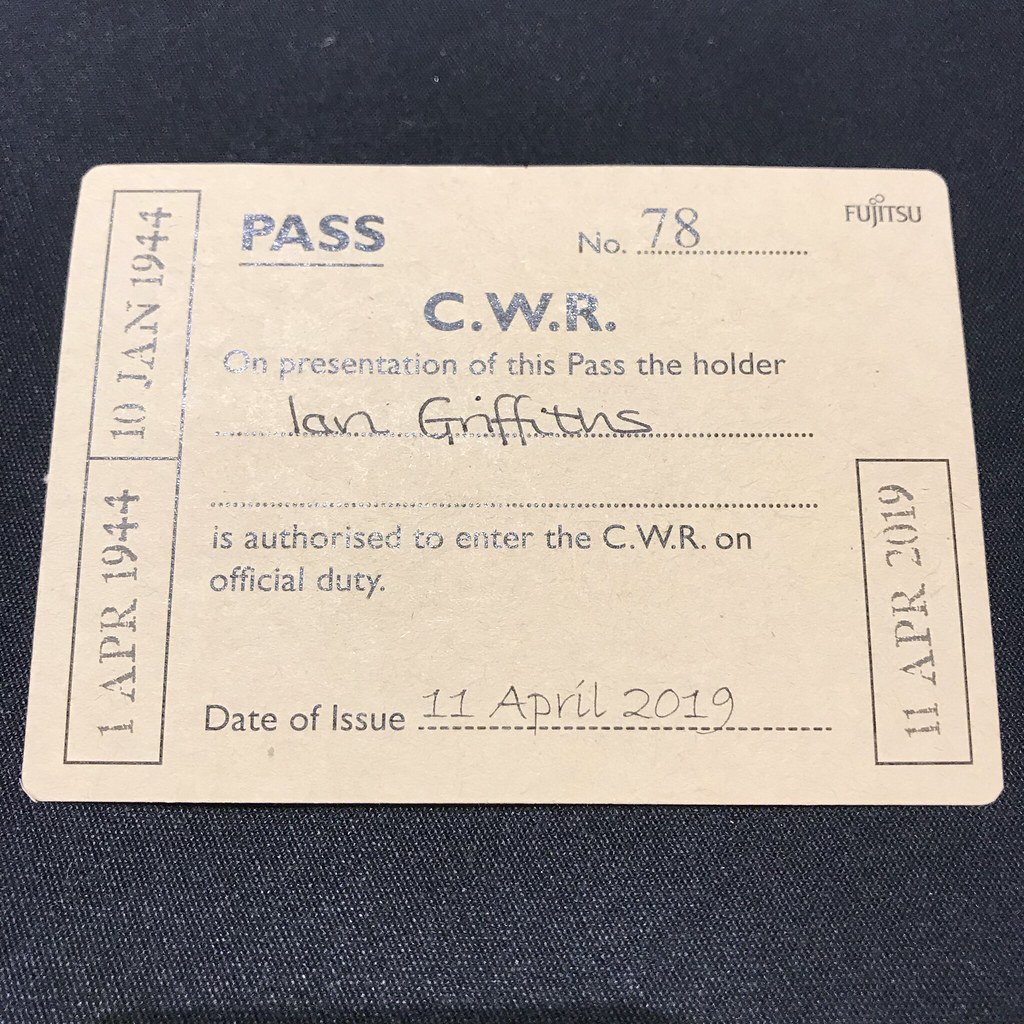This is a photograph of an off-yellow, rounded rectangle-shaped entry pass assigned to Ian Griffiths. The pass is placed on a black fabric surface with occasional thin white threads. The top center of the pass has "PASS" written in bold black letters, followed by "Number 78". The top right features the company name "Fujitsu" and "C.W.R." (with periods between the letters). The key text on the pass states: "On presentation of this pass, the holder Ian Griffiths is authorized to enter the CWR on official duty", with the date of issue being "11 April 2019" prominently displayed. Additionally, the left side of the pass displays dates "1 April 1944" and "10 Jan 1944" vertically in two stacked boxes. The pass bears a stamp or printing noting "11 April 2019" on the lower right.